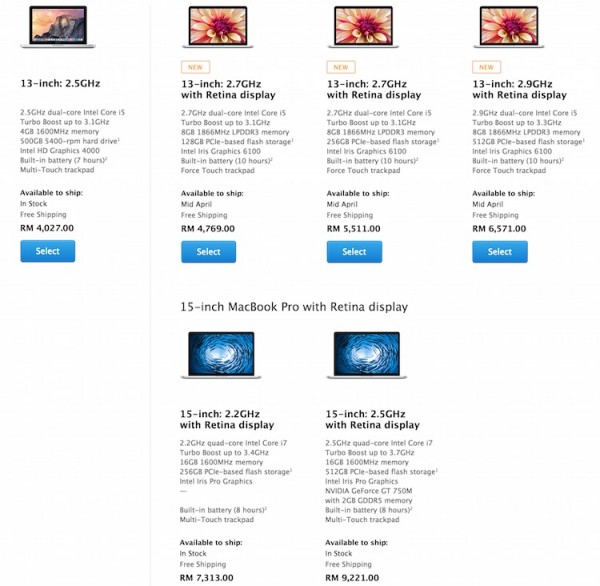The image displays a selection of computer monitors and MacBook Pro laptops with various specifications and prices. 

- The first monitor is listed as a 13-inch model with a 2.5 gigahertz processor, priced at $4,027. There is a "Select" button beneath it.
- The second monitor is a 13-inch model with a 2.7 gigahertz processor and a retina display, marked as "new" and priced at $4,769.
- The third monitor is another 13-inch model with a 2.7 gigahertz processor and a retina display, also labeled "new," but priced higher at $5,511, with a "Select" button available.
- The fourth monitor is a 13-inch model with a 2.9 gigahertz processor, featuring a retina display, and is new as well. It is priced at $6,571.

Following these monitors, there is a section for 15-inch MacBook Pro laptops with retina displays:
- The first 15-inch model has a 2.2 gigahertz processor and is priced at $7,113.
- The second 15-inch model has a more robust 2.5 gigahertz processor, priced significantly higher at $9,221.

Each item is displayed with its respective specifications and prices, along with "Select" buttons where applicable.